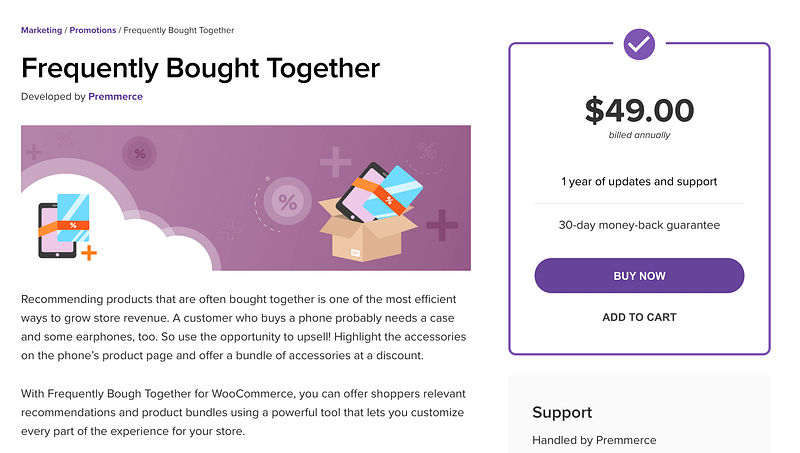This image is a screenshot of a marketing product page, presumably from an online commerce site, though the exact website name is not visible. The highlighted section is titled "Frequently Bought Together," developed by a company named Premmerce. The page features an animated illustration that includes a tablet, a card, and a plus symbol situated within a cloud. Adjacent to this is another graphic depicting a cardboard box containing the tablet and card, accompanied by a percentage sign and two plus symbols.

The caption beneath these images explains that recommending products frequently bought together is an effective strategy to boost store revenue. For instance, a customer purchasing a phone might also need a case and earphones, presenting a prime opportunity for upselling. The feature highlights accessories on the product page and offers discounts on bundled items.

The product, "Frequently Bought Together for WooCommerce," allows store owners to provide relevant recommendations and customizable product bundles. It is priced at $49 per year, which includes one year of updates and support, along with a 30-day money-back guarantee. The page also includes options to "Buy Now" or "Add to Cart," as well as a support section managed by Premmerce.